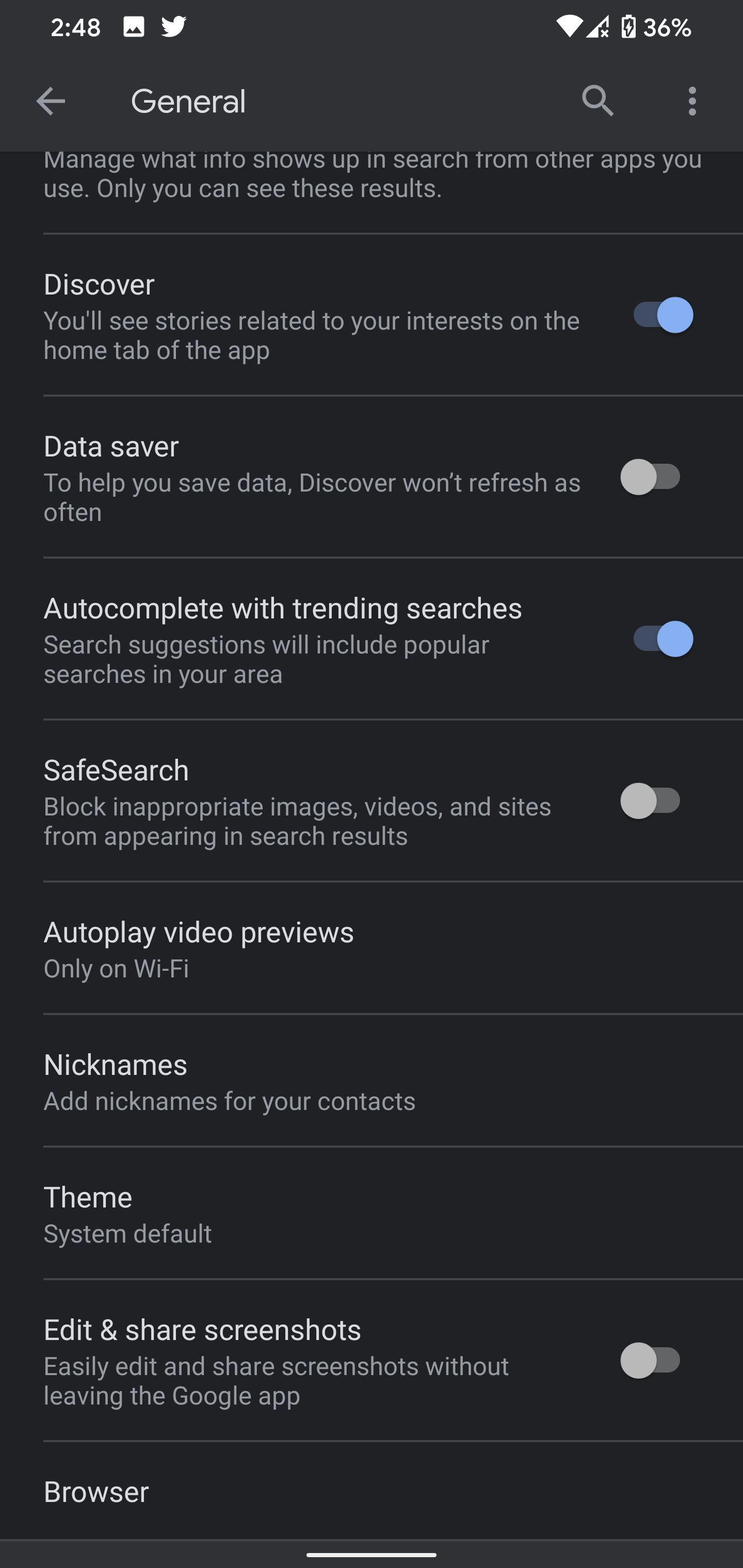The image depicts a screenshot taken from a mobile phone. The entire background is black. At the top of the screen, the time reads "2:48" and the battery is at 36%. Additionally, the status bar shows the text "General" accompanied by a left-pointing arrow on the left, a magnifying glass icon on the right, and three vertical dots aligned on the far right.

Below the status bar, various settings are listed down the screen:

1. "Discover": Indicates that stories related to the user's interests will appear on the home tab of the app. This feature is turned on.
2. "Data Saver": Mentioned as a way to help save data by reducing the frequency of Discover refreshes. This feature is turned off.
3. "Auto Complete with Trending Searches": Enabled to suggest trending searches while typing. This feature is turned on.
4. "Safe Search": This setting is turned off.
5. "Autoplay Video Previews": Configured to autoplay video previews only when connected to Wi-Fi.
6. "Nicknames": Allows users to add nicknames for their contacts.
7. "Theme": Set to "System Default."
8. "Edit and Share Screenshots": This feature is turned off.
9. "Browser": The specific settings or status for the browser are not detailed.

Overall, the image provides a detailed overview of the phone's current settings within a specific application or system configuration screen.